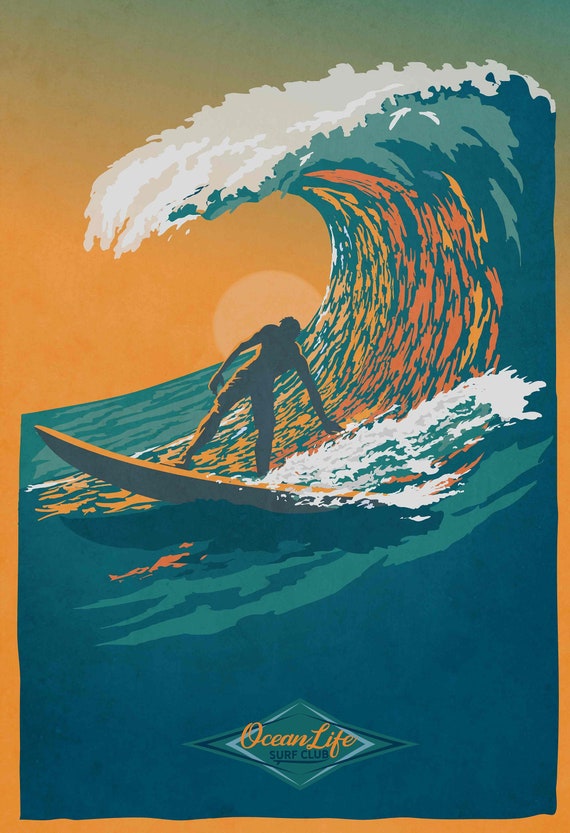The image is a detailed illustration of a surfer riding a massive wave during sunset. The style is cartoon-like, emphasizing both warm and cool colors, predominantly orange and blue. The large wave curves dramatically, almost swallowing the sun, which casts its orange reflection within the wave. The top of the wave froths with white, and splashes are created where the surfer, whose silhouette is facing away from us, touches the water with his hand. This act of surfing creates a dynamic white splash. The background transitions beautifully from an orange sky at the horizon to a blue gradient as it rises. At the bottom of the illustration, a sideways diamond-shaped logo reads "Ocean Life Surf Club." The overall scene captures the thrilling essence of surfing combined with the tranquil beauty of a sunset.